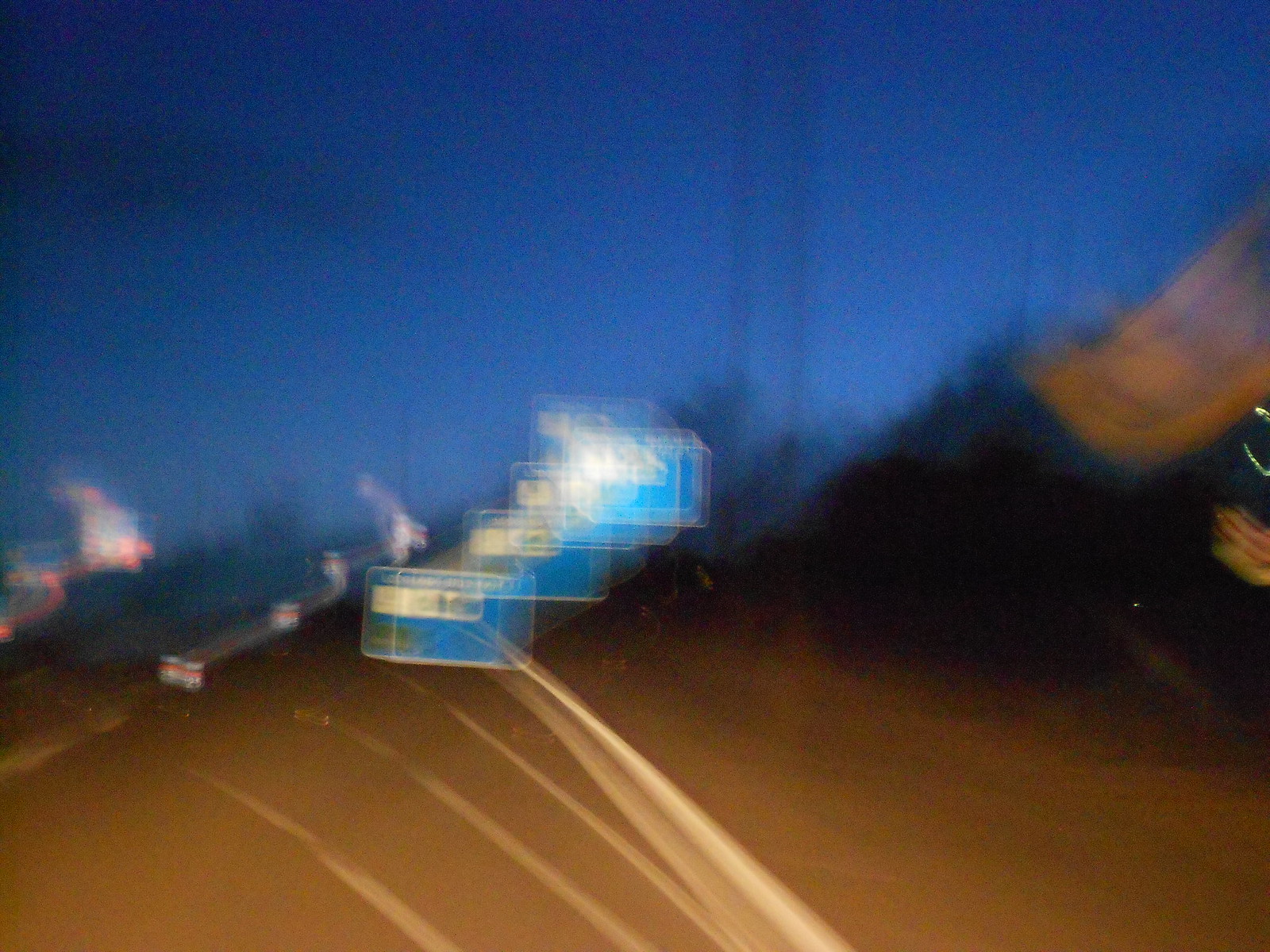This image, though blurred, appears to capture a scene taking place during the twilight hour, just as night begins to settle in. The sky retains a faint blue hue indicative of the approaching night, with an overall clear atmosphere despite the lack of sharpness in the photo. At the center of the image is what appears to be a card, possibly resembling a social security card, though it is surrounded by multiple afterimages, making it difficult to discern its exact details. To the side of the card, there is a distinct black puff or smudge. Additionally, a streak of blurred motion extends from the bottom of the image to a point near the card, suggesting swift movement occurred during the capture of this photograph.